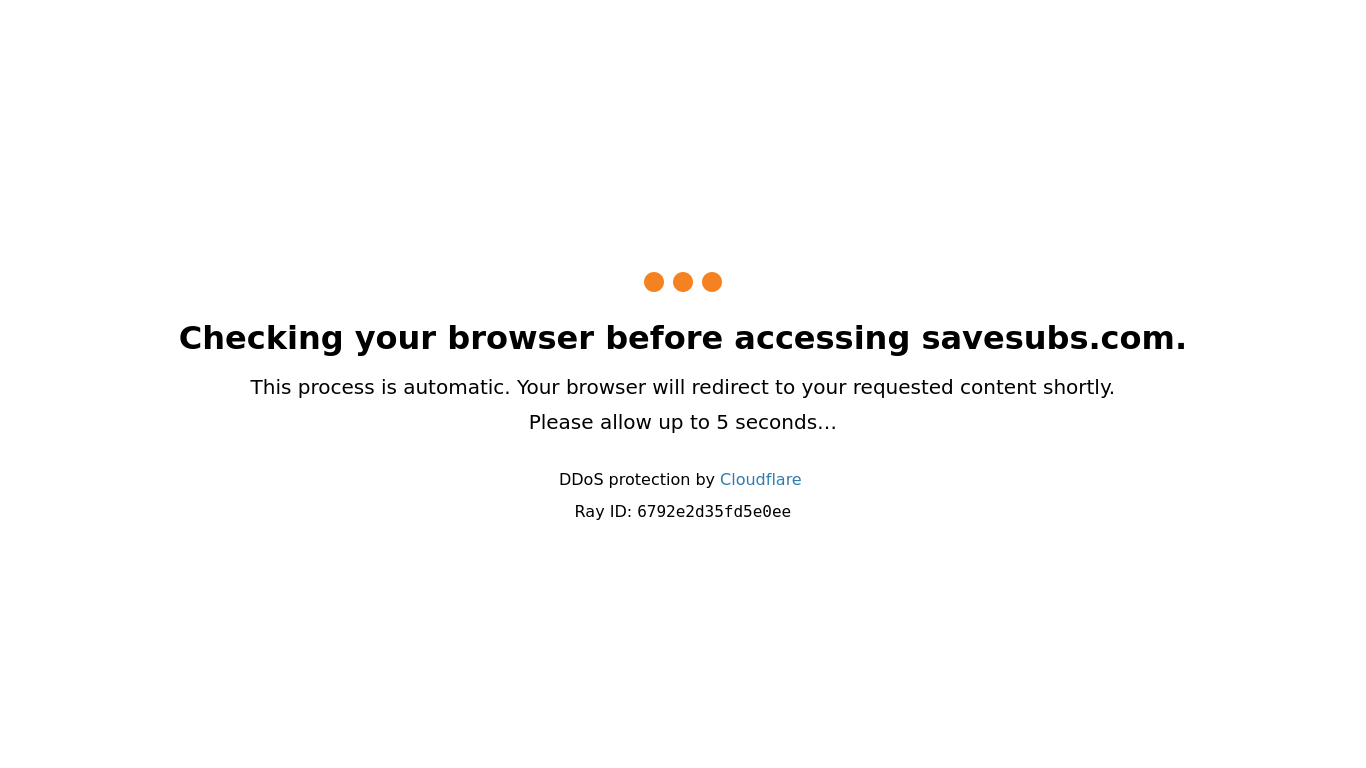**Caption:**

The image has a clean, all-white background with centered alignment. At the top middle of the image are three orange dots arranged horizontally. Below this, in the largest bold font, the text reads, "Checking your browser before accessing save subs calm." In much smaller font, the subsequent line states, "This process is automatic. Your browser will redirect to your requested content shortly." Below that, it advises, "Allow up to five seconds…" Following this, the text "DDoS protection by Cloudflare" is displayed in blue. Further down, a unique identifier "Ray ID: 6792E2D35FD5E0EE" is listed. The primary colors used in the image are white, black, orange, and blue, with no outlines or borders, giving it a seamless appearance that blends into the device's screen background. There are no indicators suggesting whether the device is a cellphone, tablet, or computer, apart from the mention of Cloudflare's protection.